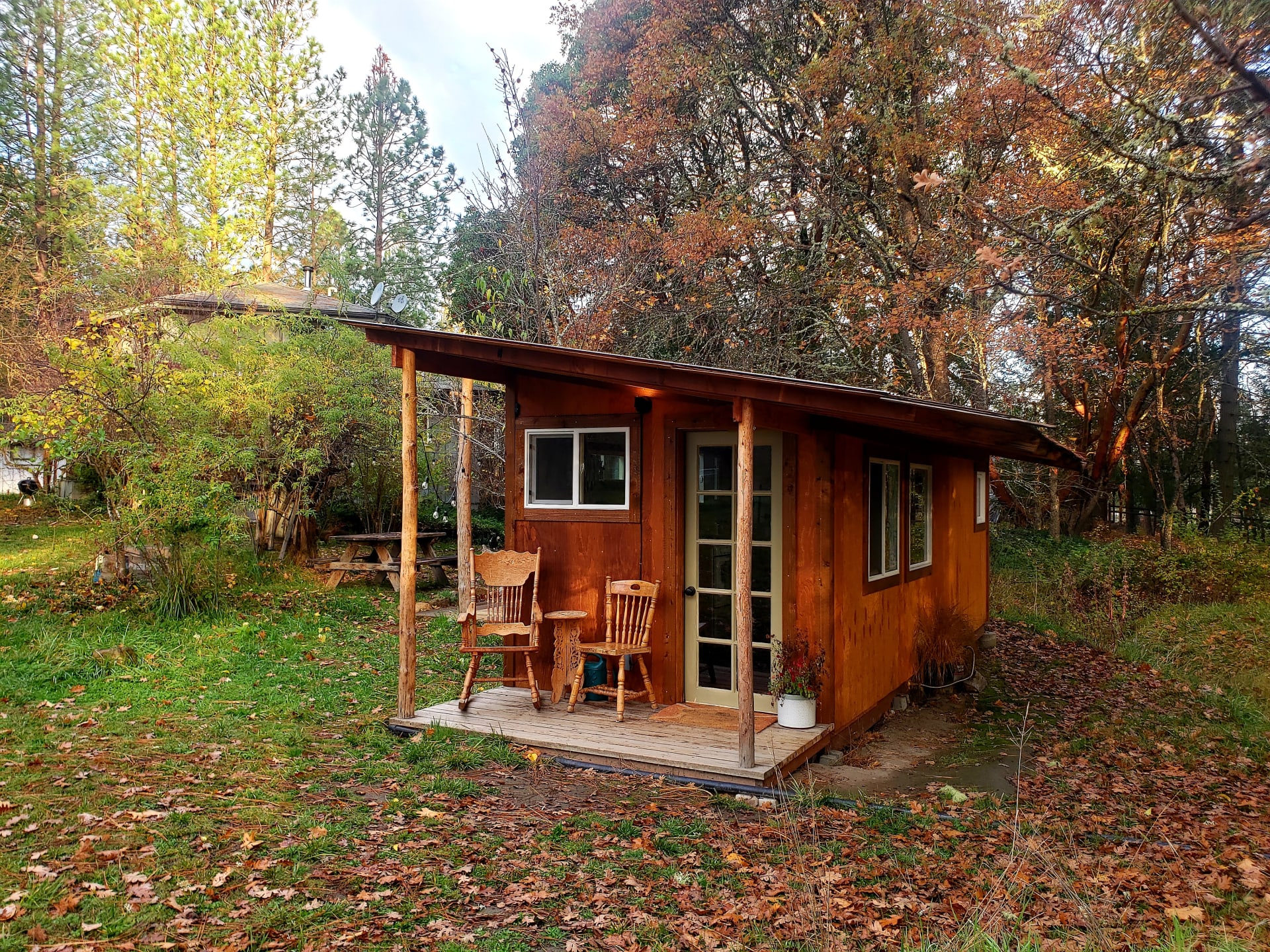The image captures a well-lit outdoor scene featuring a small, wooden structure that most resembles a cabin with elements of a shed or playhouse. This picturesque cabin is surrounded by a dense collection of trees, creating a secluded atmosphere. The cabin is equipped with a covered porch supported by wooden pillars and topped with a sideways metal roof. On the porch, there are two chairs—a rocking chair and a regular chair—set up around a small table, and a potted plant beside a doormat at the front door, which features glass panes. 

Adjacent to the cabin on the left, there are bushes and a nearby picnic table, with hints of another house roof peeking out from behind the foliage. In the distance, there is a separate structure hosting a grill. The ground is covered with leaves, indicating an autumn setting, underscored by the colorful fall foliage visible in the trees. Blue, cloudy skies peek through the tree canopy, enhancing the tranquil, rustic setting.